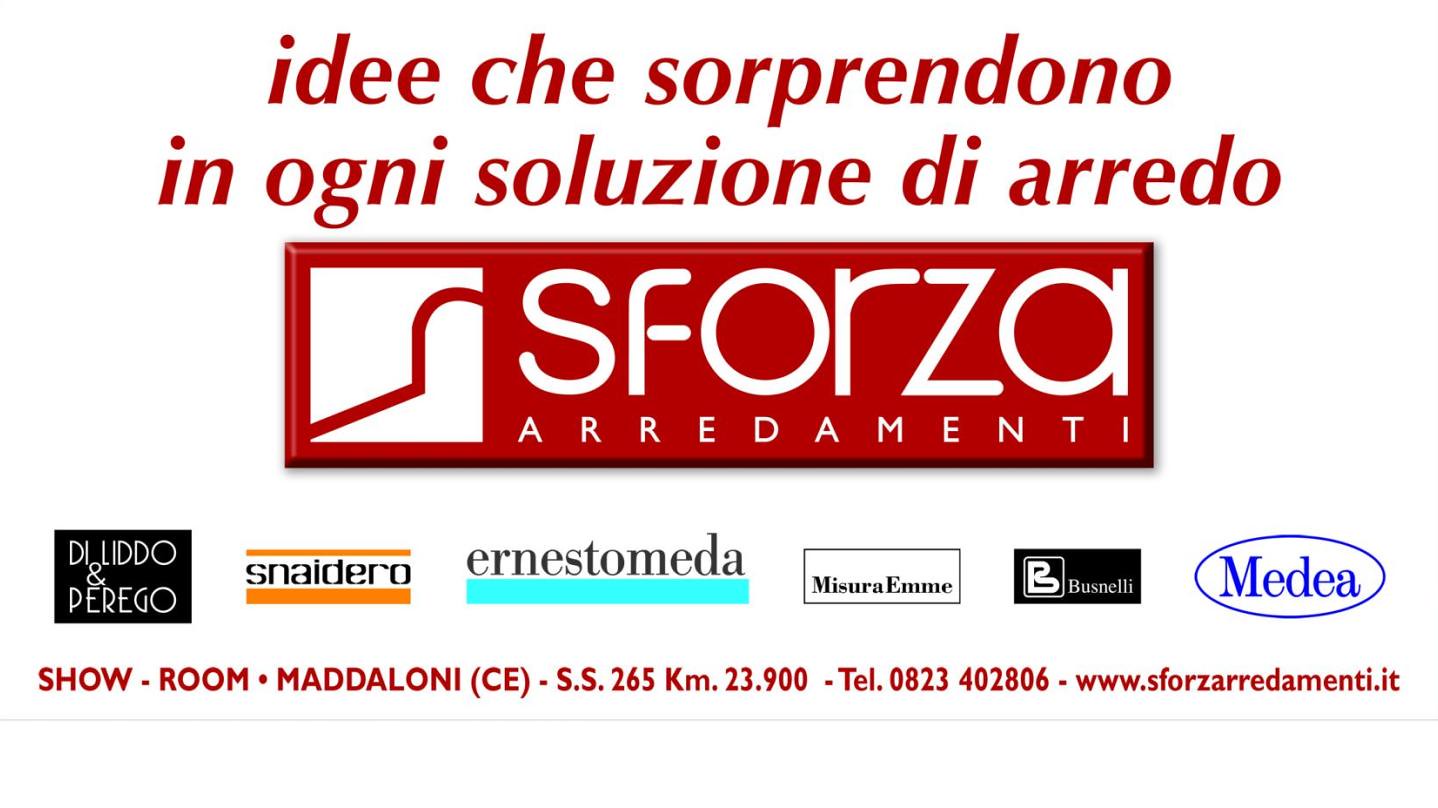The image is a wide rectangular advertisement with a completely white background. At the top, it features large italicized bold red text in Italian that reads "Idee che sorprendono in ogni soluzione di arredo." Below this, there is a wide red rectangle shaded on the sides to create a 3D effect, resembling a red brick. On the left side of the rectangle, there is a white square with a red line curving and hooking to the right, designed to look like a door in a wall. Across the red part of the rectangle, the brand name "S-F-O-R-Z-A" is written in large white text, followed by "arredamenti" in smaller justified white text. Beneath this, there are six logos for various companies. At the very bottom of the advertisement, there is contact information in small red print, including the address "Showroom Madaloni (CE) S.S. 265 km 23.900" and telephone number "0823 402806." The website "www.sforzaarredamenti.it" is also listed.